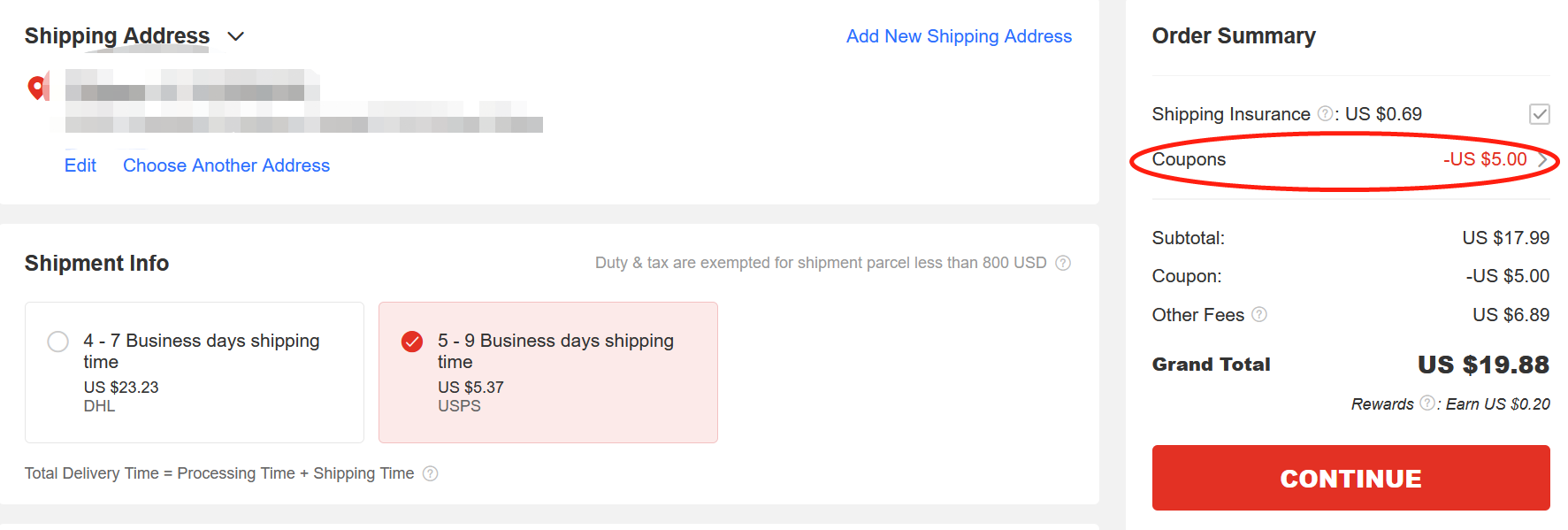The image depicts a detailed order confirmation section of a website. In the upper left corner, there is a heading labeled "Shipping Address," accompanied by a map icon and pointer. The specific name and location information are pixelated for privacy. To the right of this section, there is a blue text link labeled "Add New Shipping Address," though it appears as plain text rather than a clickable button.

Below the shipping address, there is an option to "Edit" or "Choose Another Address." Further down, shipment information is displayed with two selectable options. The first option indicates "4-7 shipping days, U.S. $2323, via DHL," and the second option, highlighted with a pink background and a red check mark, shows "5-9 shipping days, U.S. $537, via USPS." Additional details mention the total delivery time, processing time, shipping time, and note that duties and taxes are exempted for shipping parcels valued over $800.

To the right of the shipping information, in a separate column, there is an "Order Summary." This section details the breakdown of costs: shipping insurance priced at $20.69, a coupon discount circled in red showing a deduction of $5, a subtotal of $1799 minus the $5 coupon, other fees totaling $6.89, leading to a grand total of $1988. Additionally, rewards amounting to $0.20 are indicated.

At the bottom of the order summary, there is a large red rectangular button with white capital letters that read "CONTINUE."